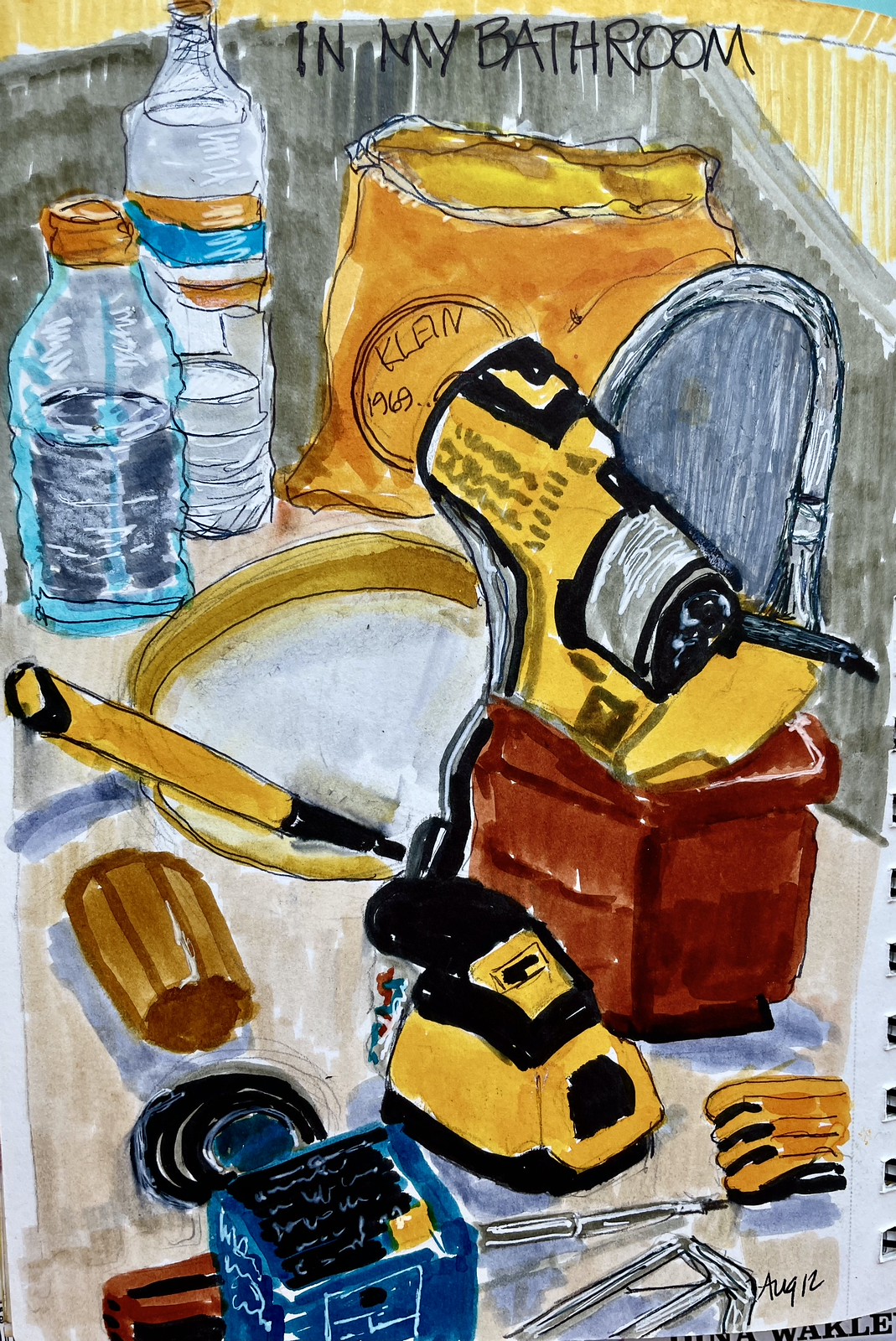The image is a detailed, hand-drawn watercolor illustration titled "In My Bathroom," printed in black font at the top. The artwork features a cluttered bathtub or sink counter environment with various items meticulously depicted. On the left side, there are two bottles with orange tops; one appears to be a water bottle and the other a sports drink with blue liquid inside. To the right of these bottles is an orange bag with a circle in the middle that reads "Climb." Below this bag, we see a red bag containing a yellow and black cordless drill, and next to it is a yellow pencil or brush, a yellow and black tape measure, and a few scattered articles such as a pen and possibly a ruler. Towards the back, there is a sink with a faucet, and in the sink, a yellow-handled brush or small tool. The white countertop also holds a yellow Dewalt vibrating sander, a leather glove, and more assorted tools including a screwdriver and an allen key set. Off to the right, there's the wire binding of the artist's notepad, and at the bottom, the date "Aug 12" is written in script. The detailed depiction captures a chaotic yet familiar scene, reminiscent of a busy workbench placed in an unusual bathroom setting.